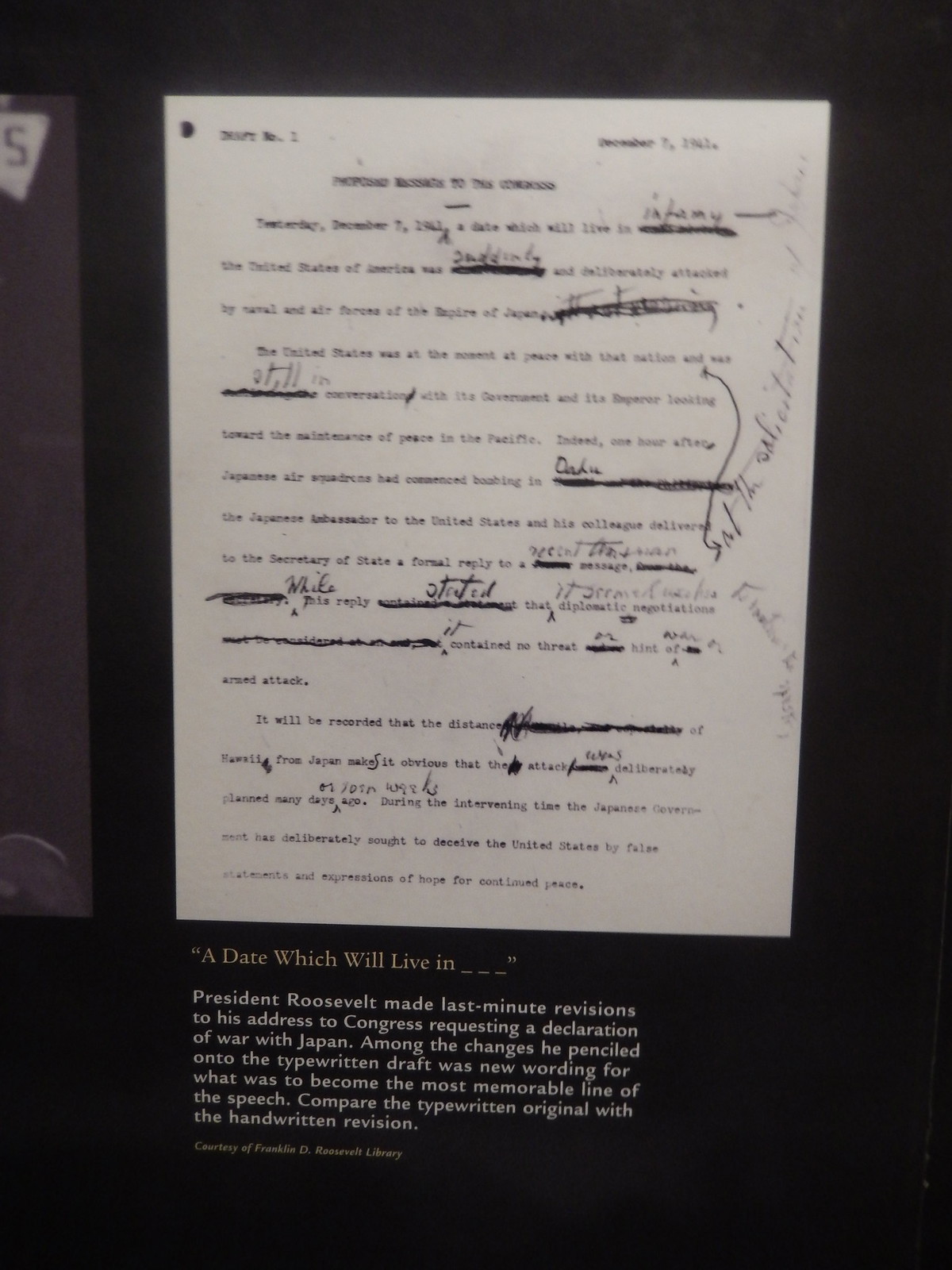Displayed against a black background, the image features a blurry, old-fashioned memo with numerous parts crossed out and various edits written in pen. The letter, likely drafted by President Roosevelt before his historic address to Congress requesting a declaration of war against Japan, is a typewritten document with handwritten revisions. The most notable alteration includes the rephrased line that would become the iconic "a date which will live in infamy," distinguished in a goldish color, while the rest of the text appears in white. Below the memo, printed letters spell out a caption about President Roosevelt's revisions, memorializing this pivotal moment in history. The poor image quality suggests it might be a photograph from a museum exhibit documenting Roosevelt's last-minute changes.